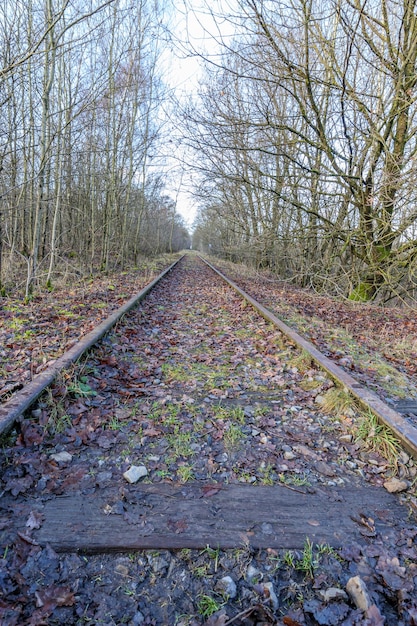This image captures a disused railway track running through a barren woodland area. The photo is taken from the perspective of someone standing directly on the track, looking down. Dead leaves cover the ground beneath, and the tracks themselves are slightly rusted, with a single wooden plank visible amidst debris. The surrounding trees are leafless, emphasizing a desolate, perhaps late fall or very early spring setting. The overall ambiance is dull and brown, with bright green moss on some trees hinting at emerging growth. A light, overcast sky adds to the somber, wet and potentially rainy atmosphere of the scene. Sparse patches of green grass are pushing through the leaf-littered ground, signaling the cusp of seasonal change.